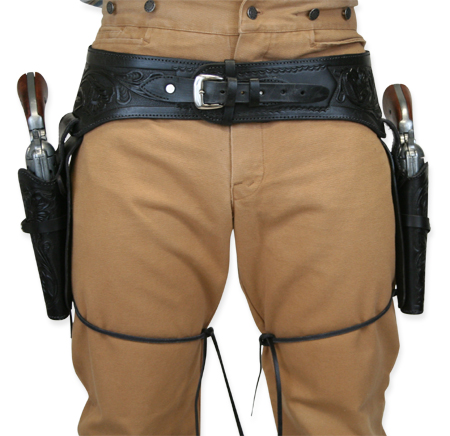The photograph showcases a detailed view of a cowboy's attire from slightly above the knees to the middle of the abdomen, set against a plain white background, emphasizing the subject. He is dressed in light brown or tan jeans with five round buttons visible and wears a black, decorated leather belt with a silver buckle in the front. On either side of his hips, two black leather holsters hang, each containing a pistol with shiny metal bodies and brown wooden grips featuring silver trim. The holsters are secured to his legs with thin black strings tied just above the knees, ensuring they stay in place, a feature not commonly seen. The intricate details of the western wear, including the silver rivets and the functional design of the dual holsters, contribute to the authentic cowboy look, completed by the "western O" marking found in the upper part of the image.